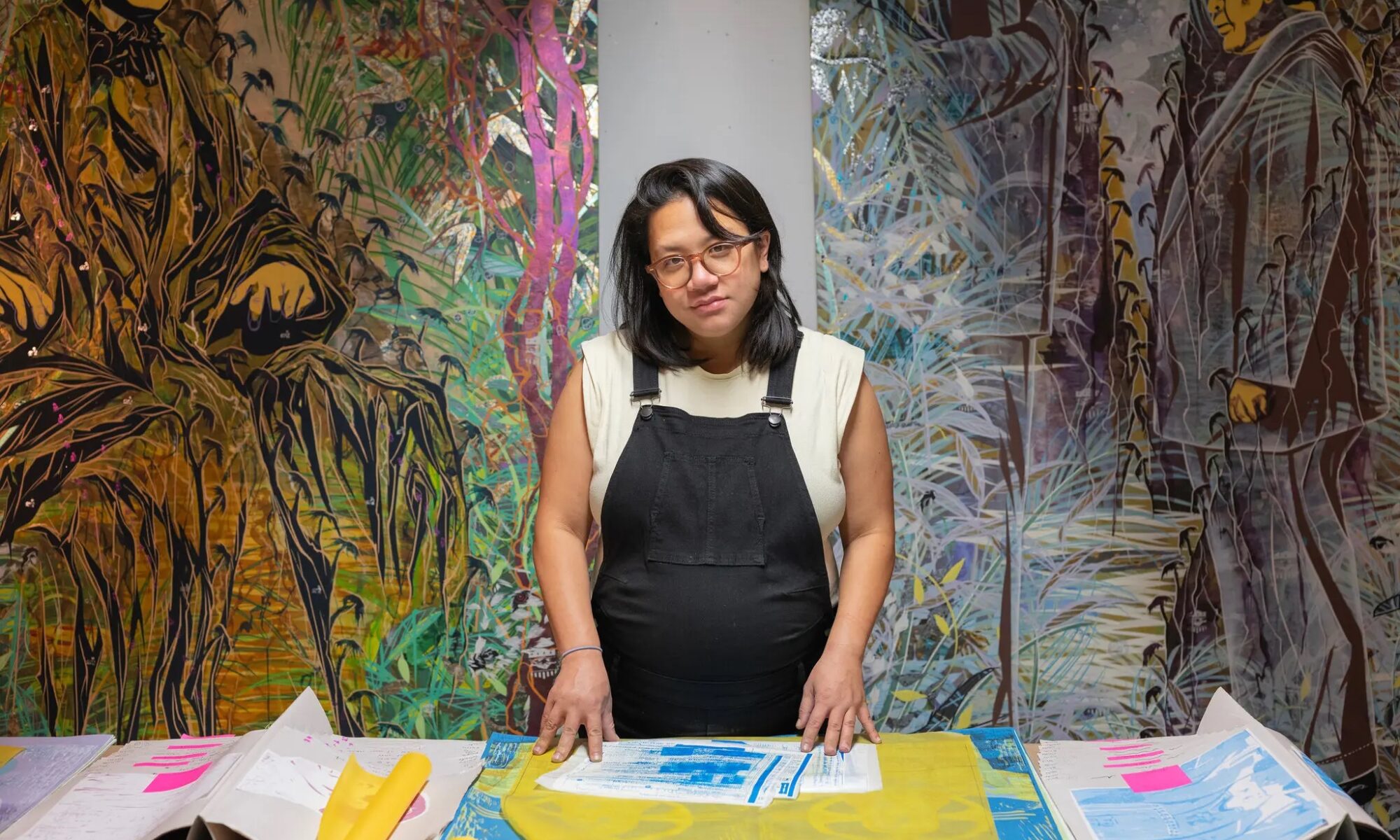This photograph captures a woman in a studio, standing centered amidst an artistic backdrop. On either side of her, impressionistic paintings adorn the wall; to the left, a yellow-tinged painting depicts a man in a robe seated, while to the right, a bluish painting portrays a man in a large suit standing and facing left. The bottom of the frame features a table cluttered with various paintings and papers: a white piece with pink rectangles on the left, a blue and yellow painted piece in the center, and another smudged blue and pink rectangular piece on the right. The woman, possibly of Filipino descent and of average build, has long black hair cascading past her shoulders and wears pink-rimmed glasses. Dressed in black overalls and a white sleeveless shirt, she gazes directly at the camera, her hands resting on the blue and yellow paper in front of her, with a hair tie on her wrist. Behind her, the wall is rich with abstract art and vibrant colors, creating an immersive, creative atmosphere.